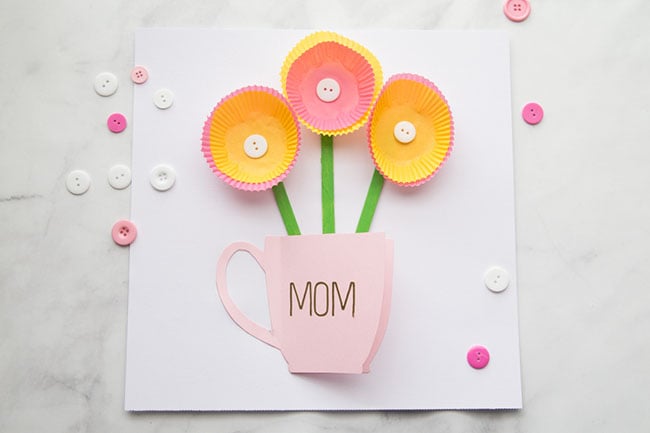This is a detailed photograph of a handmade Mother's Day card crafted by a child. The image is set against a white marble background. The central focus is a square white sheet of paper. At the bottom center of the sheet, there is a pink paper mug with the word "Mom" written on it. Emerging from the top of the mug are three green paper stems, representing flower stalks. Each stem is topped with cupcake liner flowers: the two outer flowers have pink liners on the bottom with orange liners on top, while the middle flower features a yellow liner on the bottom and a pink liner on top. All three flowers have white buttons glued at their centers, mimicking flower pollen. Scattered around the sheet and the marble surface are assorted pink and white buttons, adding to the whimsical and festive appearance of the craft, as if capturing the creative process in action. The overall presentation is reminiscent of a child's heartfelt artistic effort, celebrating their mother in a simple yet charming manner.